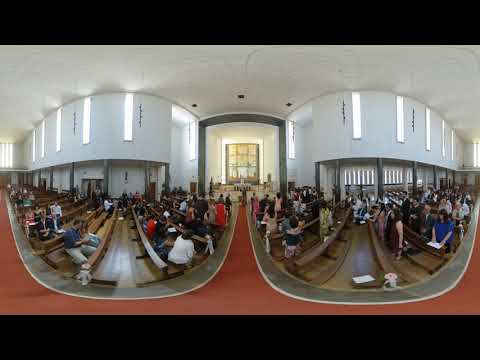This is a panoramic collage, a 360-degree photograph seamlessly stitched together, capturing the interior of a modern church. The horizontally aligned image, framed with thick black borders at the top and bottom, features two prominent circular areas that create an optical illusion resembling the lenses of eyeglasses. These circular shapes effectively segment the view into two halves, each showcasing different sections of the church.

On the left, we see congregants seated in wooden pews, with a few individuals standing. On the right, another group of people faces towards the pulpit, also seated in pews. Both halves are connected by a central aisle covered in red carpeting, which visually forms a 'W' shape as it diverges towards two groups of pews. This red aisle leads directly to the altar, where a detailed stained glass window can be seen.

The church interior is bright, illuminated by white lights and narrow vertical windows that line the upper sections of its white walls, contributing to a modern aesthetic. The overall architecture is not particularly traditional, featuring elements that hint at a contemporary design. Despite the distorted lines and skewed perspective typical of a 360-degree shot, the image offers a compelling and comprehensive view of the church’s layout, including its vibrant community and architectural details.